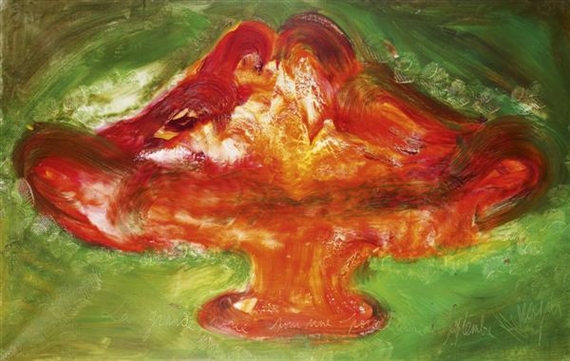This abstract painting features a central red, blobbish form reminiscent of lips or a mouth, but it also evokes the imagery of a mushroom, tongue, or flower, with a viscous, almost melting quality. The red dominates the piece, accented by streaks of yellow and white speckles, particularly on the left side and center. The reddish object appears to be melting into a puddle at the bottom, anchored by rounded edges and a pedestal-like base. The painting's green background, punctuated with dark green and white blotches, provides a stark contrast. The upper right corner is a darker green, offering depth, while thick, bold brushstrokes add texture and movement. A signature, scratched into the bottom right corner, remains illegible.